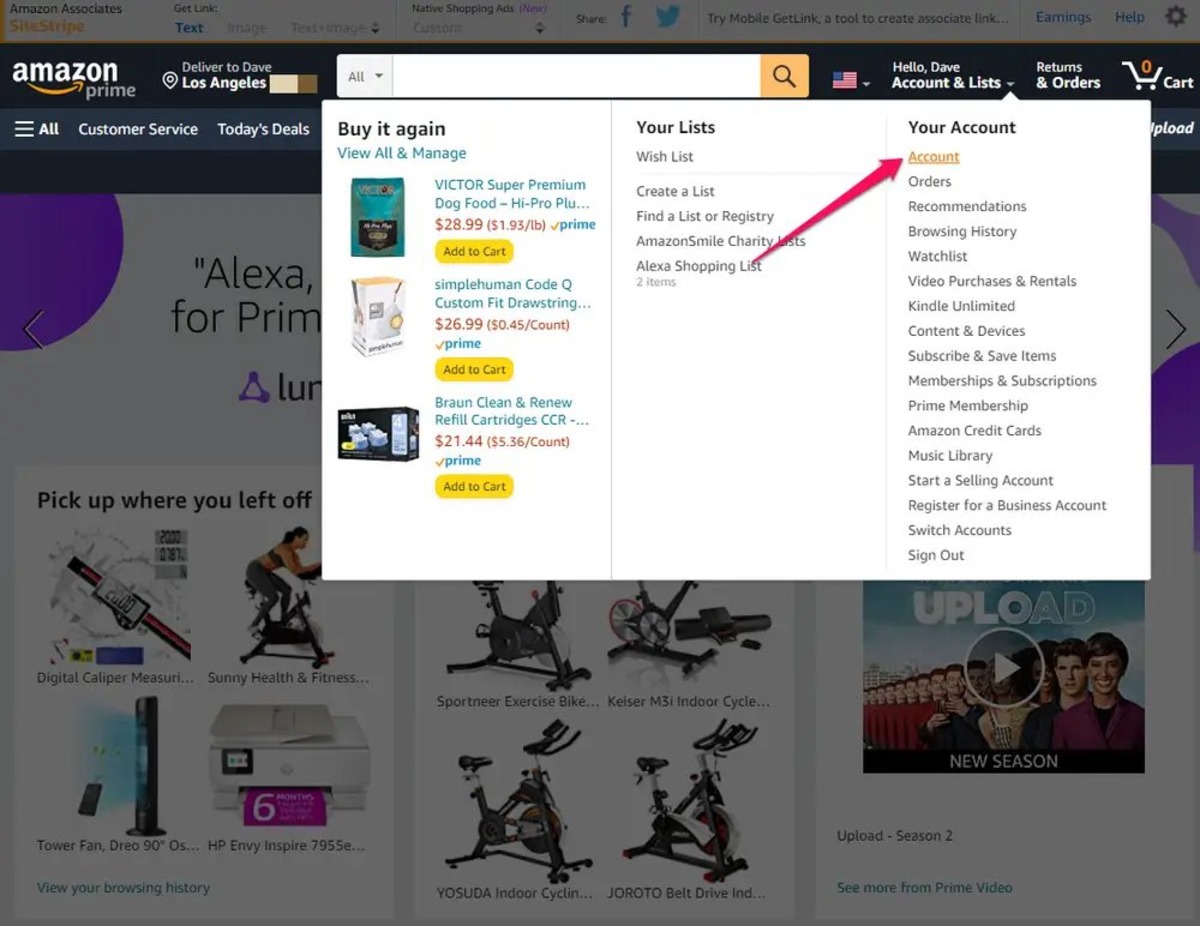This image captures the Amazon website, with a user, Dave, actively signed into their account. The distinctive Amazon logo, featuring a white font with a signature yellow smile and arrow, is prominently displayed in the top left corner on a dark blue banner that spans the width of the screen. This banner also showcases the word "Prime" in a gray font.

Above the main banner, a grayed-out white section hosts various informational links such as "Amazon Associates," "Get Link," "Text," "Image," "Text + Image," "Native Shopping Ads," as well as sharing options for Facebook and Twitter. This section also includes links for "Try Mobile," "Get Link," a tool for creating associate links, "Earnings," "Help," and a settings cog icon.

Beneath the top banner, the user’s delivery information is partially visible with their name and city (Los Angeles) shown, though the zip code is blurred out for privacy. The central dark blue banner contains a search box flanked by options like "Buy Again," "Your List," and "Your Account." Dave has opened a dropdown menu, which appears as a white box with black and gray text. This dropdown, positioned just right of the search bar, greets the user with "Hello, Dave," and provides quick access to "Account" and "List" management.

To the far right of the banner, options for "Returns & Orders" are available, with a cart icon indicating zero items in Dave’s shopping cart. The background of the homepage is grayed out due to the open dropdown menu, but it still reveals various product listings and Prime Video offerings on the right-hand side, along with advertisements at the top.

This detailed depiction of the Amazon homepage offers a comprehensive view of the user interface, highlighting Dave’s personalized account details and the website's navigational features.